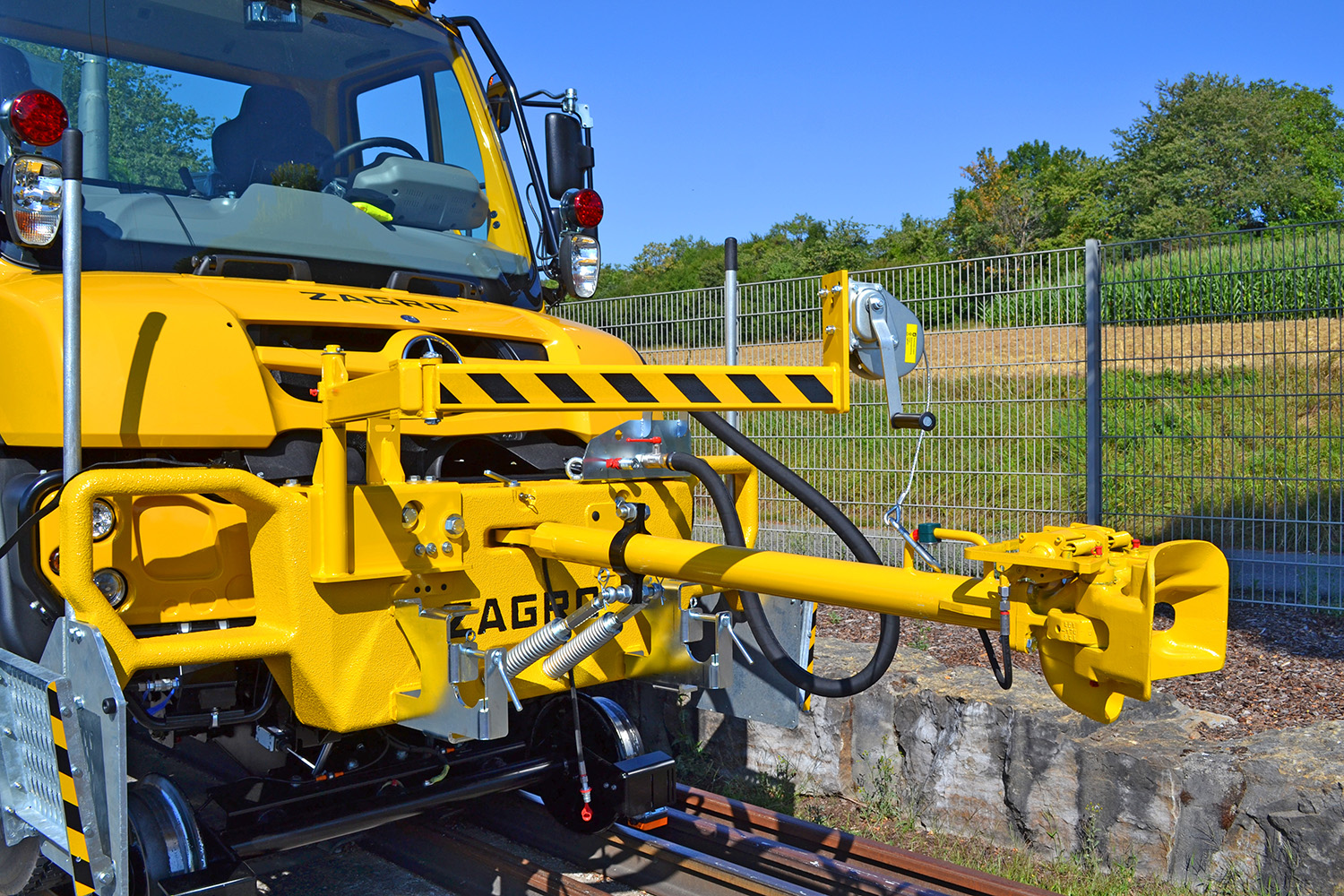A photograph captured outdoors during a sunny day, featuring a vibrant yellow construction vehicle, likely a railroad maintenance truck. Positioned on dark brown metal railway tracks, the truck displays silver metal wheels fitting precisely over the tracks. The front section of the vehicle showcases a prominent metal panel decorated with black diagonal stripes, and near the grill, an attached metal tube with a coupling for connecting to other railway cars. ‘ZAGRO’ is emblazoned in black letters across the front hood and bumper. The cockpit area has a large transparent windshield revealing the driver's seat and steering wheel, though it is unoccupied. Additional features include two red headlights on either side and a small pulley near the front. The scene is set against a backdrop of a rocky ledge, fenced with metal railing, and a sloped hillside covered with green grass and trees under a clear blue sky.